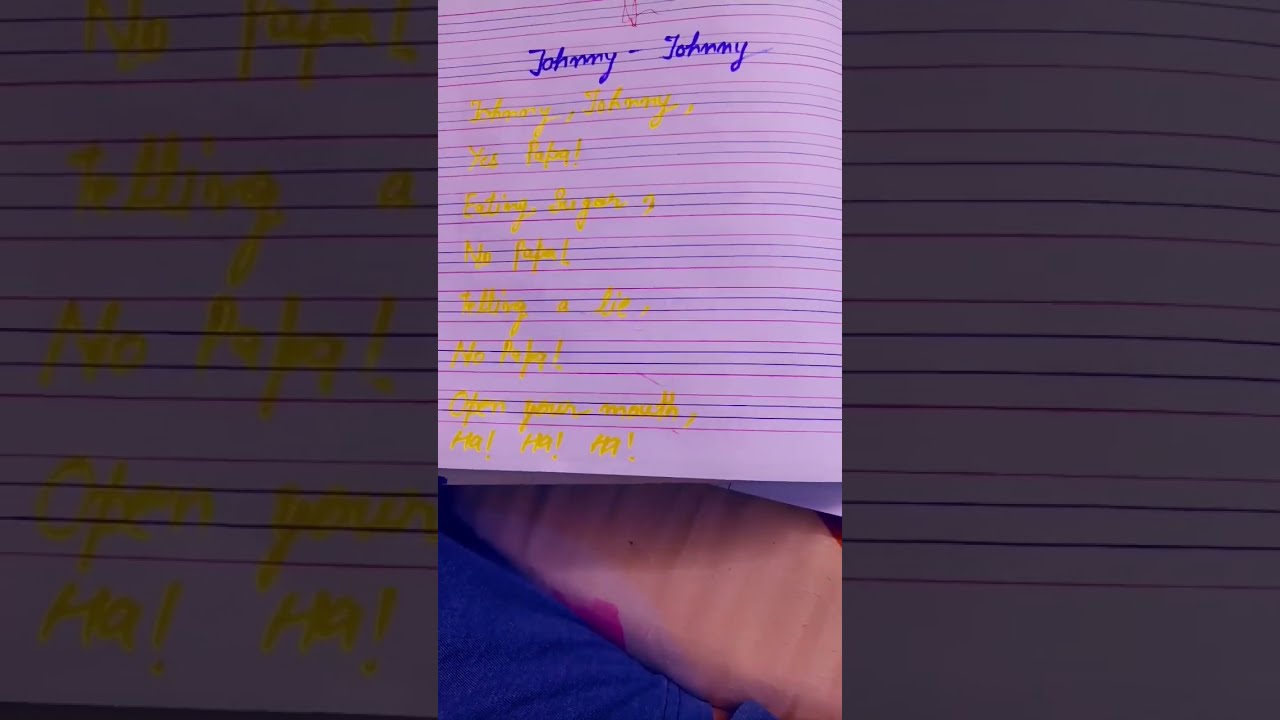In this image, there's a notebook prominently positioned towards the top of the frame, which appears to be captured in an indoor setting, potentially on a bed or couch. The notebook is distinguished by lavender-colored paper with lines that are purple and blue. The most noticeable inscription on the notebook is the repeated use of the name "Johnny" written in blue ink at the top, followed by more occurrences of "Johnny" and additional unreadable words written in yellow ink, resembling song lyrics. The final line of text consists of "ha ha ha" and "no ha", all punctuated with exclamation points. At the very top of the notebook, there is a red square scribble. Beneath the notebook lies some brown fabric with pink or red accents, as well as a patch of medium blue fabric. The colors throughout the image include blue, tan, pink, purple, yellow, and off-white, adding a vibrant mix to the scene.